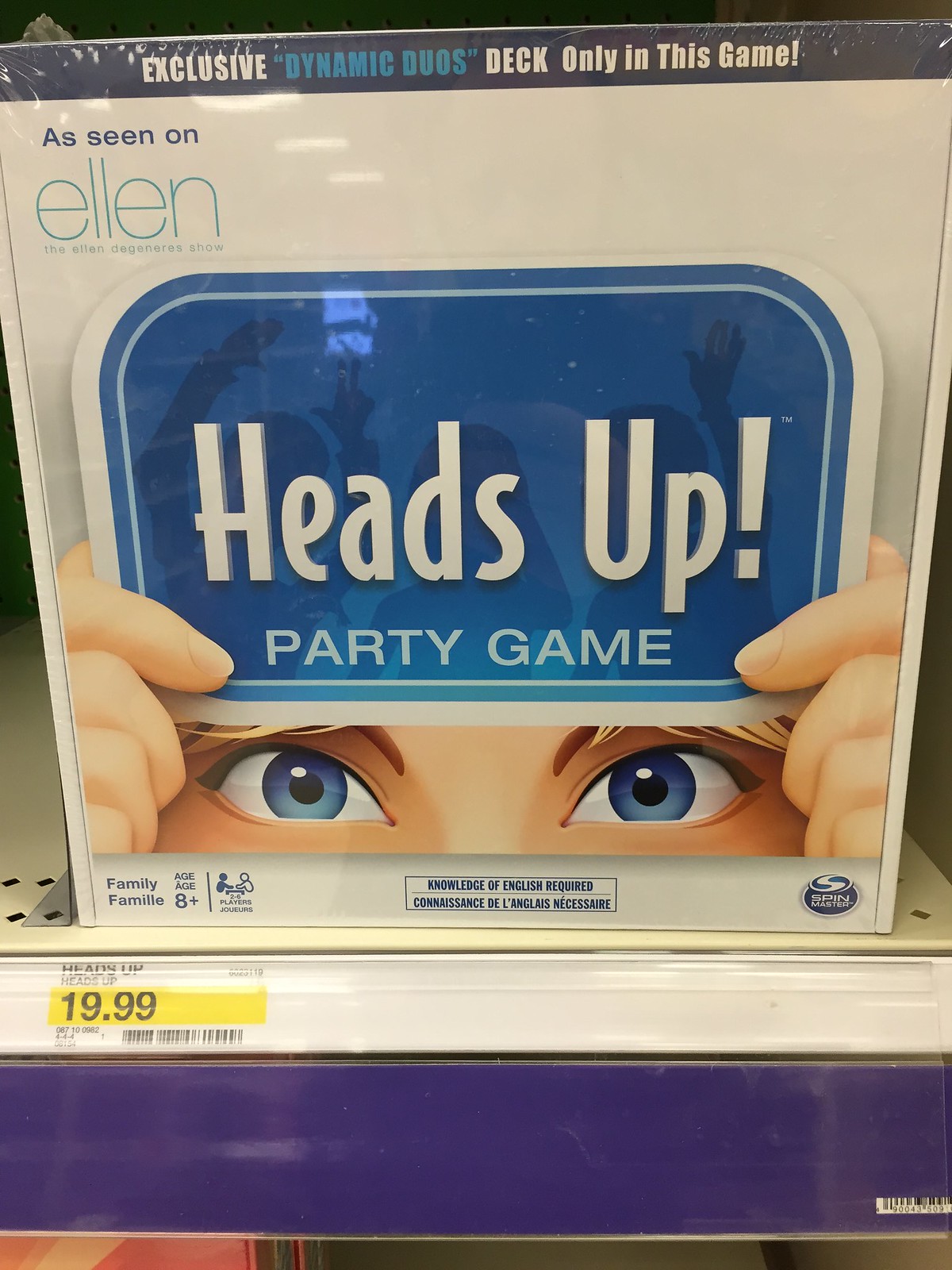The photograph is a close-up of a product on a brightly lit store shelf. The product is a shrink-wrapped, white box featuring a colorful illustration of a person with blue eyes and blonde hair holding a card up to their forehead. The card reads, "Heads Up! Party Game." The top of the box displays a black bar with the text, "Exclusive Dynamic Duos Decks Only in this game, as seen on Ellen, the Ellen DeGeneres Show." The bottom of the box provides additional information: "Family, ages 8+, knowledge of English required, Spin Masters." The box sits on a white metal shelf, above a purple plastic bar, with a price tag directly below it. The tag reads "Heads Up!" along with "19.99" in black text on a yellow background.